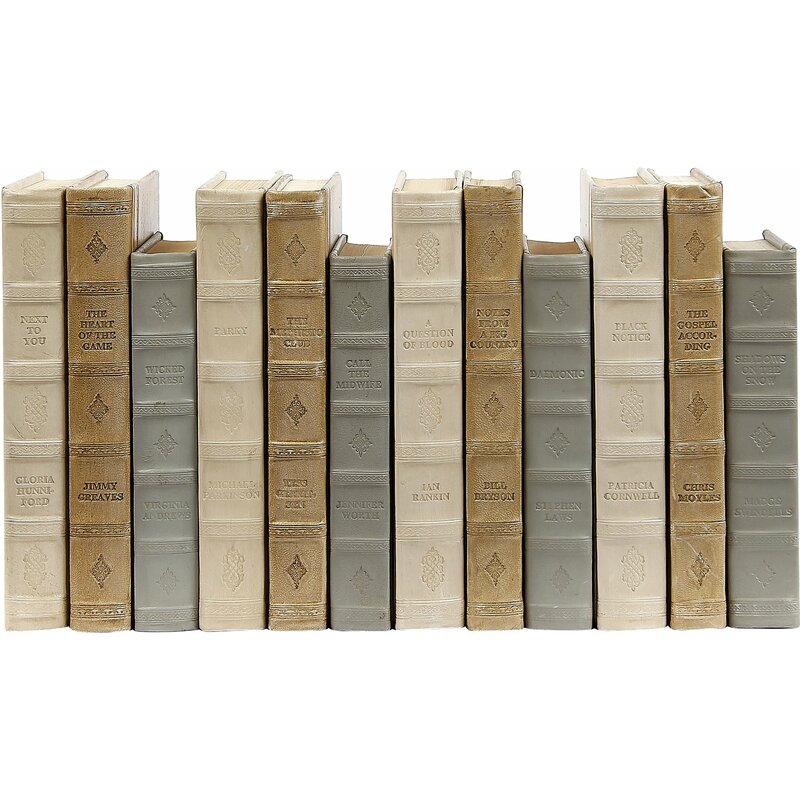The image shows a collection of 12 meticulously hand-bound books, each encased in either off-white, tan, or blue leather, exuding an old-fashioned charm. They are arranged in a repeating pattern of alternating height and color: two taller off-white and tan books followed by a shorter blue one. Each book is artfully detailed, almost giving the impression of being sculpted out of clay. The sequence of book titles includes Next to You by Gloria Hunford, The Heart of the Game by Jimmy Greaves, The Wicked Forest by Virginia Andrews, and Parky by Michael Parkinson. Other titles in the collection are Call the Midwife by Jennifer Worth, A Question of Blood by Ian Rankin, Notes from a Big Country by Bill Bryson, Demonic by Stephen Laws, Black Notice by Patricia Cornwell, The Gospel According to Chris Moyles, and Shadows on the Snow, although the last author's name is unclear. The overall arrangement creates a visually striking and cohesive display of literary works.